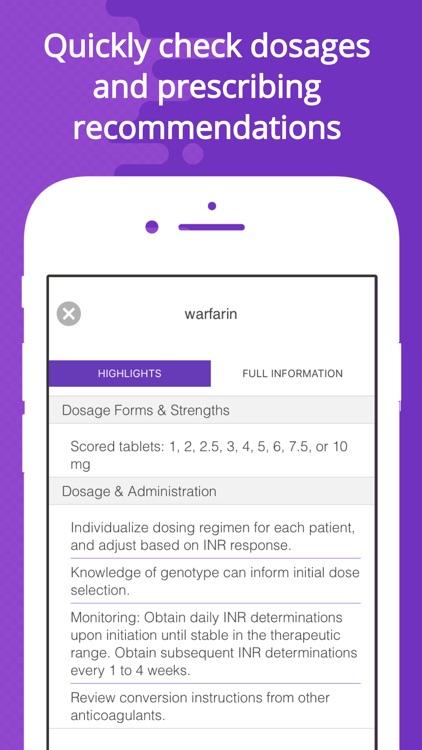This image is a screenshot taken on a cell phone displaying quality information related to doses and prescribing recommendations. The header, "Quickly Check Doses and Prescribing Recommendations," is written in white text on a purple background. Below this header, there is a clip art image of a white cell phone, not an actual device. 

The clip art cell phone features discernible side buttons on the left and a small button on the right. The screen of the cell phone showcases dosing information for prescriptions, with two selectable options at the top: "Highlights" on the left and "Full Information" on the right. The medication referenced on the phone is labeled "Warfarin" at the top of its display.

The screen further provides detailed medical dosage information, including sections such as "Forms and Strengths" and "Dosage and Administration," among others. Maintaining a consistent purple background, the white clip art cell phone stands out prominently, presenting crucial medication information in an accessible format.